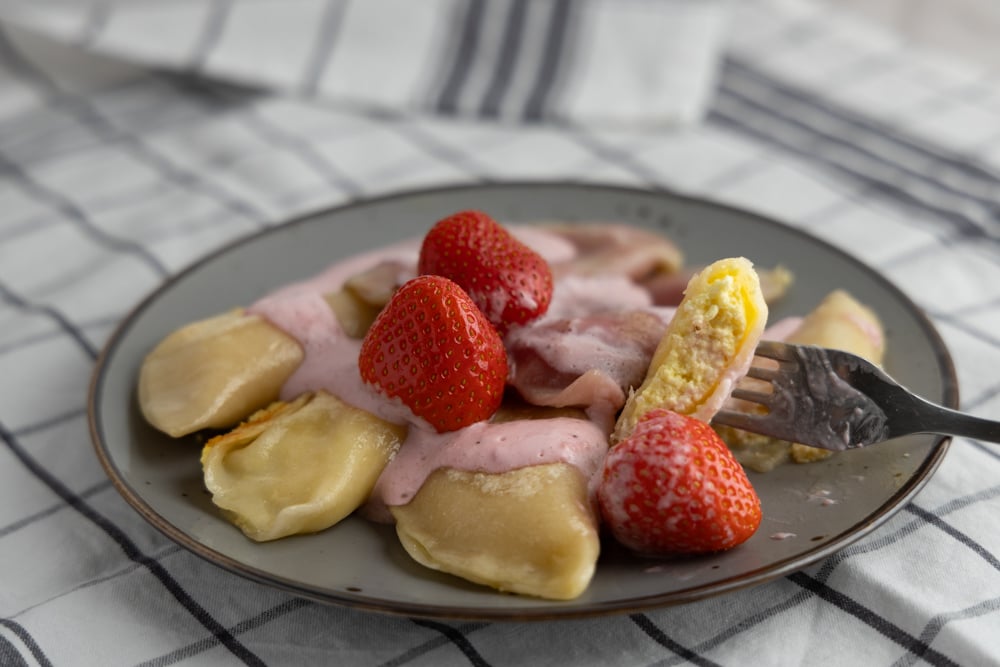The image depicts a detailed close-up of a grey plate with a brown edge, set on a white tablecloth with grey checkered lines. The focus is on the front of the plate, which features several cream-colored dumplings, some covered in a thick, pink, foamy sauce. Three whole strawberries adorn the plate, with one strawberry cut open to reveal a yellow stuffing inside. A silver fork, piercing one of the dumplings, rests on the side. In the blurred background, there are pinkish, possibly fluffy objects and hints of additional table settings, including a napkin. The captivating scene emphasizes the vibrant mix of textures and colors: the creamy pink sauce, the red strawberries, and the dumplings’ off-white and yellow hues.